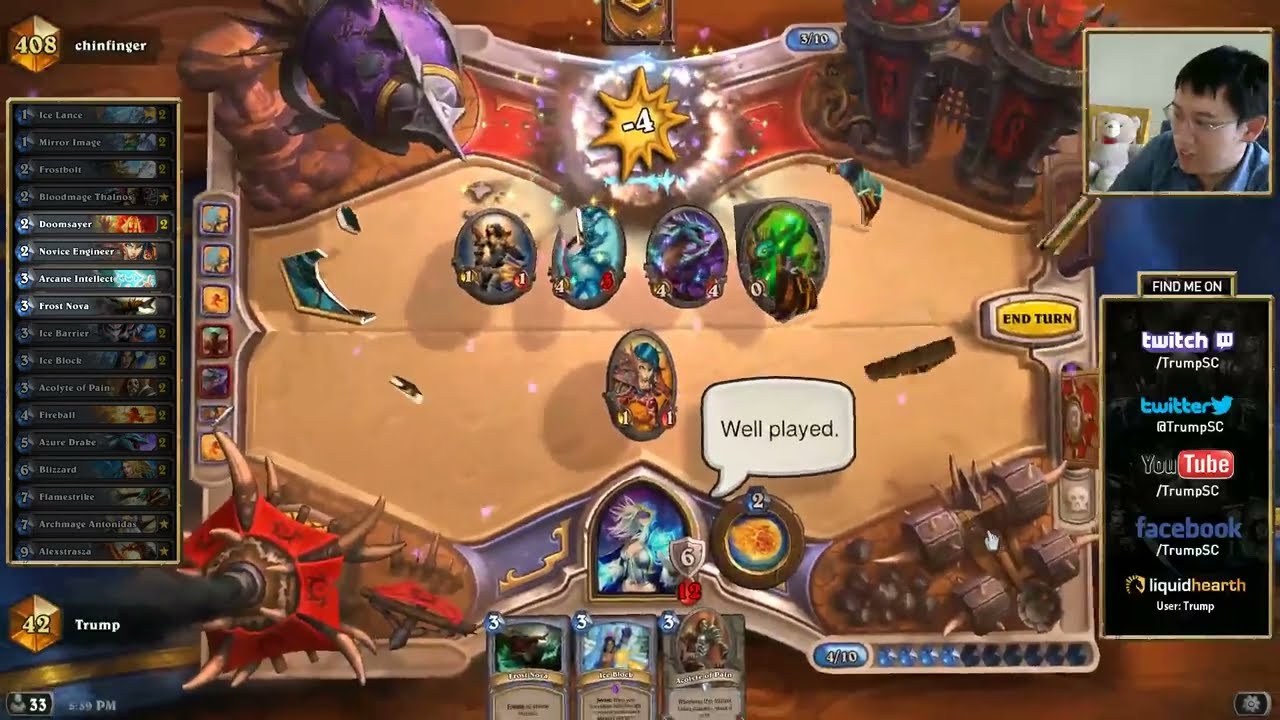This image showcases a detailed scene of a Twitch stream, where the main gameplay screen features what appears to be a fantasy-themed card game with medieval artwork and various vibrant colors, including blues, reds, yellows, browns, and purples. In the center, the game board is laid out with different cards and emblems, suggesting a strategic card-battling gameplay reminiscent of Magic: The Gathering or a Dungeons & Dragons-style game.

The top right-hand corner displays a video feed of the streamer, a young Asian man in his mid-20s, with black hair, fair skin, glasses, and a bluish-gray button-down shirt. Behind him, over his right shoulder, a gray teddy bear with a green or red bow tie is seated on a light wood-colored chair. Directly below the video feed is a box listing the streamer’s social media handles, showing his presence on Twitch, Twitter, YouTube, Facebook, and Liquid Hearth, with the handle "Trump SC."

To the left side of the screen is text related to the cards that might be in the streamer’s deck, while additional text in the main gameplay area includes phrases such as "intern Trump," indicating interaction or player status within the game. The overall lively and colorful interface reflects the engaging and strategic nature of the game being played and streamed live to an online audience.